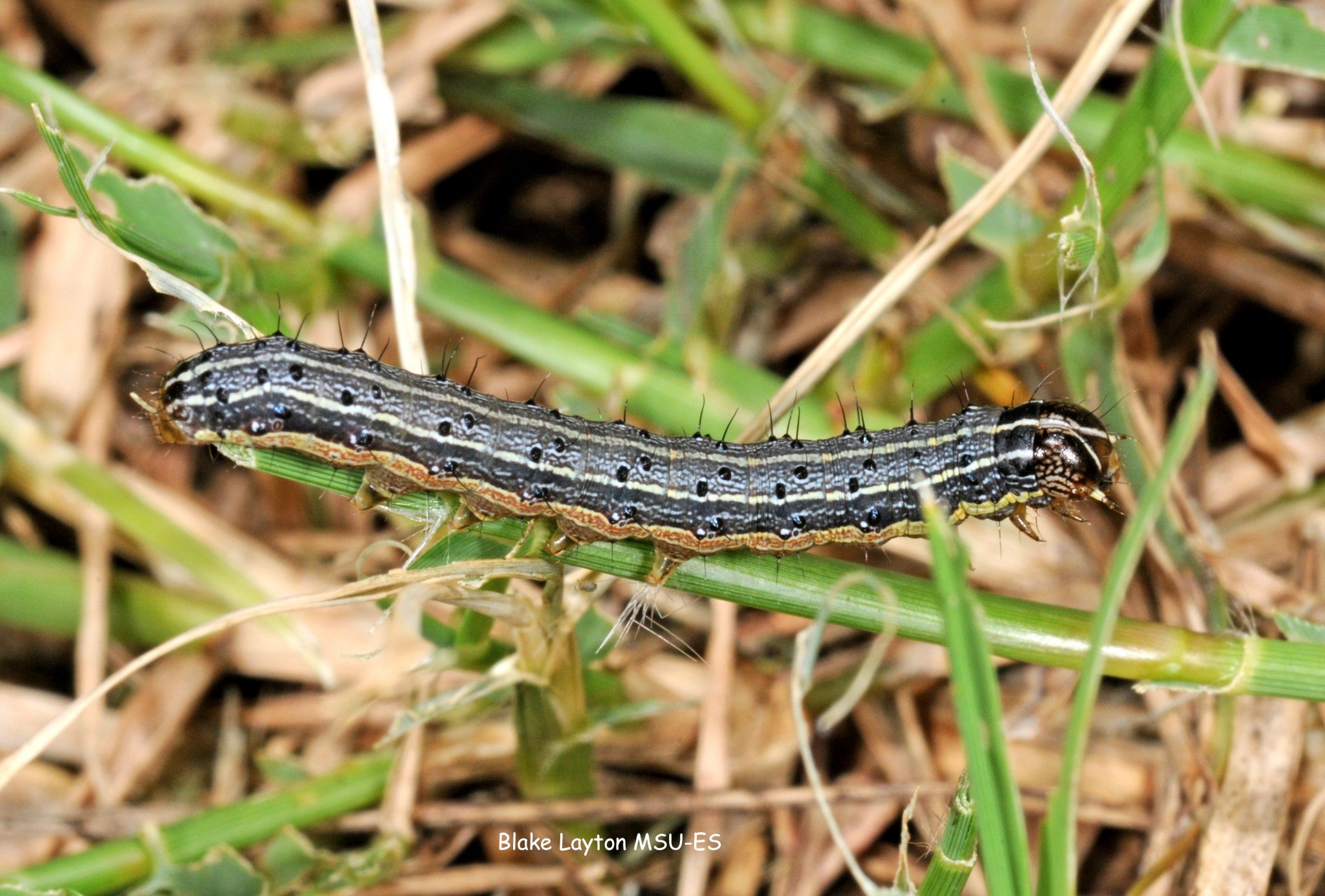This vibrant color photograph captures a detailed close-up of a long caterpillar, prominently displayed as it traverses a green stalk at the center of the image. The caterpillar, facing right with its head raised, exhibits a striking color pattern, primarily black with gold and blue stripes, white accents, and little black bumps along its body. The lower part of its body hints at yellowish and red hues. Delicate hairs adorn the caterpillar, adding texture to its segmented appearance. Tiny claws or feet are visible, gripping the stalk securely. Surrounding the creature are various green plant stems and leaves, with some wood branches and light brown mulch faintly discernible in the background. The image bears a slight blur in the background, emphasizing the caterpillar’s sharp focus. At the bottom of the photograph is a text caption that reads, "Blake Layton MSU-ES," in clear script. The overall presentation of this rectangular image delivers a detailed and vivid depiction of the caterpillar amidst its natural habitat.